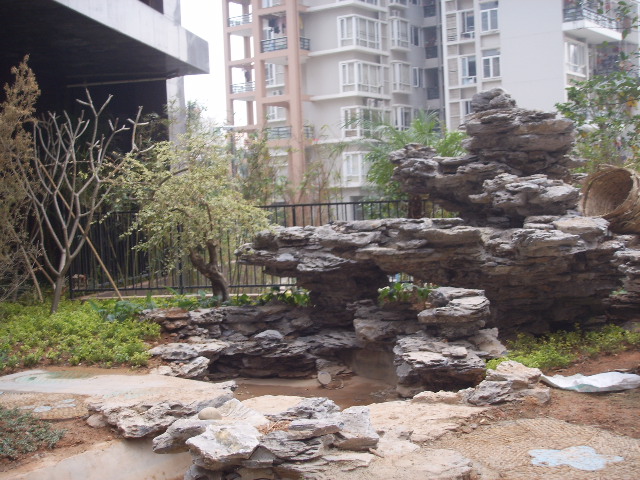This detailed color photograph captures an outdoor garden adjacent to a multi-storied apartment complex, under the daylight sky. Dominating the background is a tan, five or six-story apartment building with white-framed windows, some equipped with air conditioning units. The foreground features a sturdy black metal fence, likely demarcating the garden area. Specifically, to the left, part of a neighboring building's silver roof is visible.

The garden's centerpiece is a prominent multi-leveled rock formation, composed of tightly layered gray rocks that give the impression of having been shaped by the steady wear of water over time. Below this formation, there is a small, brownish puddle of water and a scattering of stones throughout the garden.

The peripheral greenery includes three slender ornamental trees with sparse foliage, situated above a small patch of green grass. The rest of the vegetation consists of low bushes and greenery mingled with patches of brown soil, adding a natural touch to the rocky surroundings. The garden's variety of colors – from the black of the fence to the shades of brown, gray, green, tan, white, and silver – creates a visually interesting and serene urban oasis.